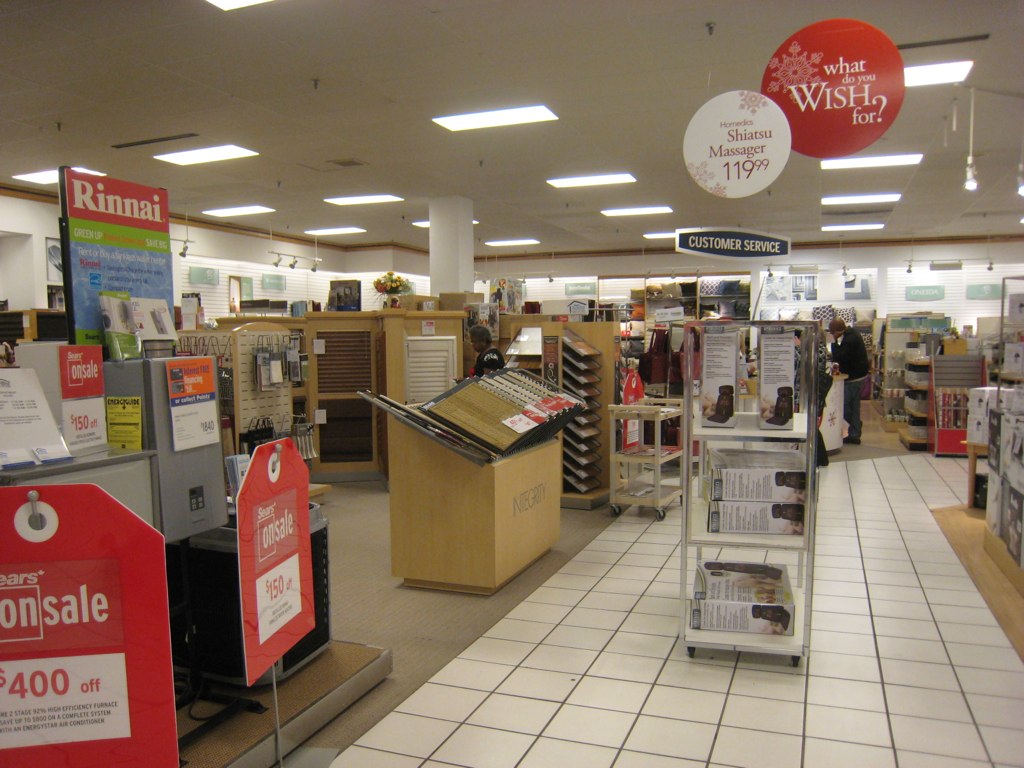This is a detailed color photograph taken inside what appears to be a Sears department store. The image captures a brightly lit aisle with various stands and shelving units, mostly constructed from wood. The floor features a mix of white tile with dark black grout and sections with beige carpet or light wood. In the foreground, there is an end cap showcasing massage chairs labeled "Satoshi Massager $119.99" with a corresponding circular sign above in purple text on a white background. There is another prominent sign hanging above that reads "Customer Service" in white text on a black background. Additionally, two eye-catching red circular signs with white text hang nearby, one of which says "What do you wish for" with a white snowflake emblem. Scattered throughout the aisle are various sale signs, including some red tags indicative of discount offers, such as "$150 off." Furniture pieces, including a table displaying wood tiling and flooring samples and possibly sample books for shutters or blinds, are lined up along the aisle. One sign reads "Rene," and in the background, a shopper dressed in a black shirt and brown pants is seen, possibly receiving assistance from customer service.